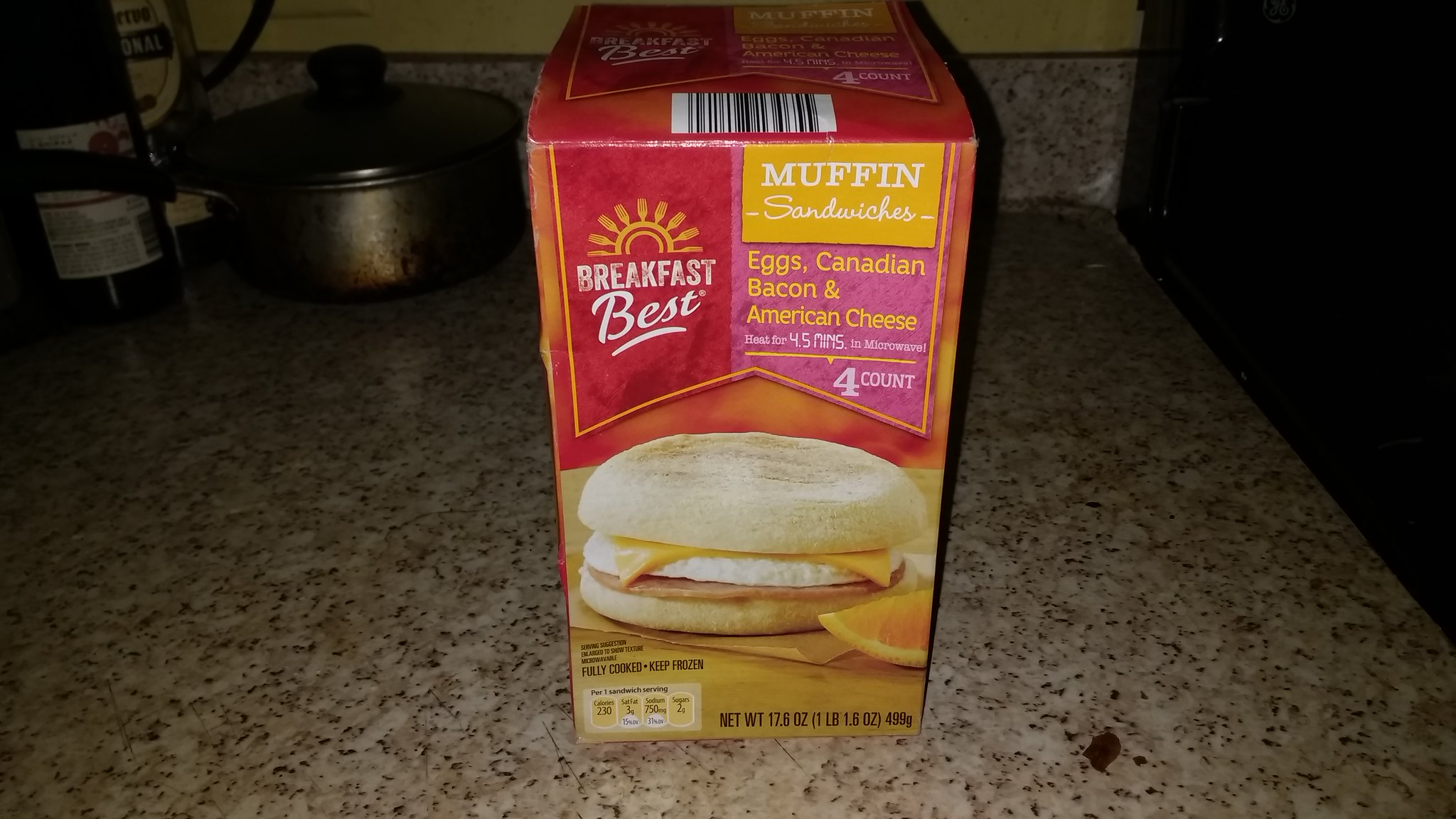The close-up photograph features a red and orange box labeled "Breakfast Best Muffin Sandwiches," prominently displayed on a tan marble countertop speckled with light brown, black, and gray. The box showcases an appetizing image of a light brown English muffin sandwich filled with egg, Canadian bacon, and American cheese. Next to the sandwich on the box, there's an orange wedge. The box also specifies a net weight of 17.6 ounces (1 pound, 1.6 ounces) and indicates that the sandwiches can be microwaved for 4.5 minutes. In the background, a silver pot with a black handle and some gray and black areas sits on the countertop, along with a red bottle with a white label. The backsplash matches the tan marble countertop, featuring spots of black, light gray, and chocolate brown. The image conveys a cozy kitchen setting, focusing on the appealing breakfast option.